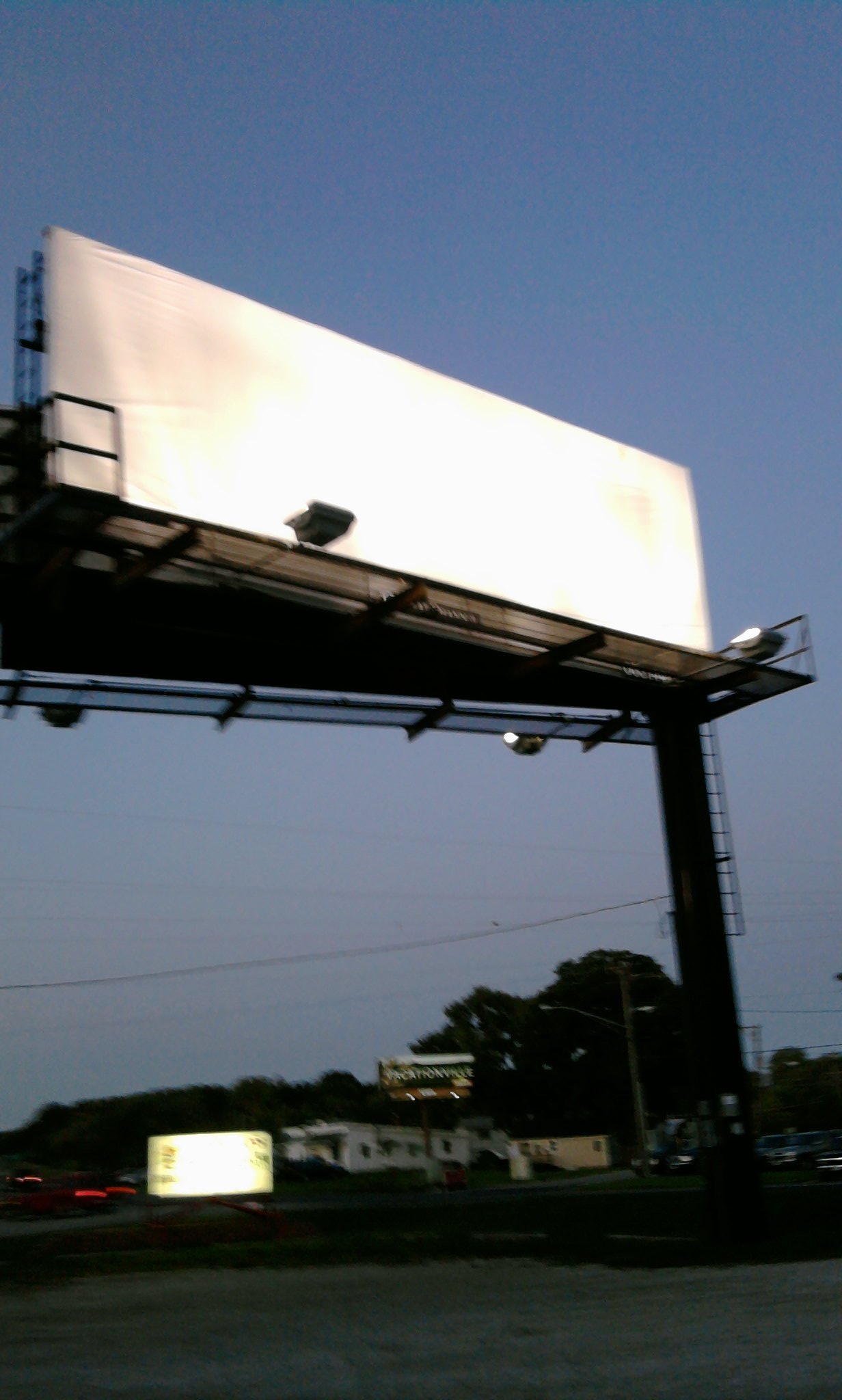The photo, taken outdoors at either dawn or dusk, features a large, rectangular billboard prominently displayed above a road. The billboard is supported by a sturdy metal foundation with a ladder and a catwalk. It is illuminated by two lights that render the billboard's surface completely white and overexposed, making any text or images on it illegible. In the foreground, part of the road is visible, suggesting the picture may have been taken from inside a vehicle due to the presence of what appears to be a reflective white square, possibly a car window. To the right of the billboard, there is a structure resembling a stairway, used to access the billboard. The background showcases a gray sky with trees and a trailer, accompanied by a smaller building and a rectangular, yellow ground-level sign that is glowing yet unreadable. Additionally, there are faint brake lights visible in the lower left-hand corner, enhancing the scene's atmospheric lighting.